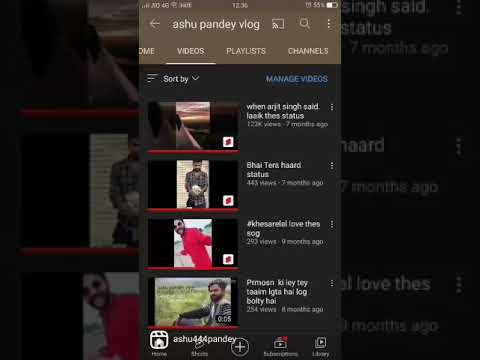This image is a detailed screenshot of the YouTube channel page for a user named Ashu Panday Vlog. At the very top, there is a status bar displaying the time as 10:42, the battery level, and various other status icons. Directly below this, a search bar prominently shows 'Ashu Panday Vlog' entered in the search field. Beneath the search bar, the page features several navigational tabs including Home, Videos, Playlist, and Channels, with the Videos tab currently selected, indicating that the list of the channel’s uploaded videos is being shown.

In the top right corner under the search bar, there is an option to manage videos indicated by a highlighted 'Manage Videos' button. The videos are organized in a vertical list format, displaying the thumbnail on the left and the video details on the right which include the video title, view count, and upload time.

The first visible video in the list is titled "When Arijit Singh Said Back Thanks," featuring a thumbnail image of a person. This video has garnered 1.2 thousand views and was uploaded 7 months ago.